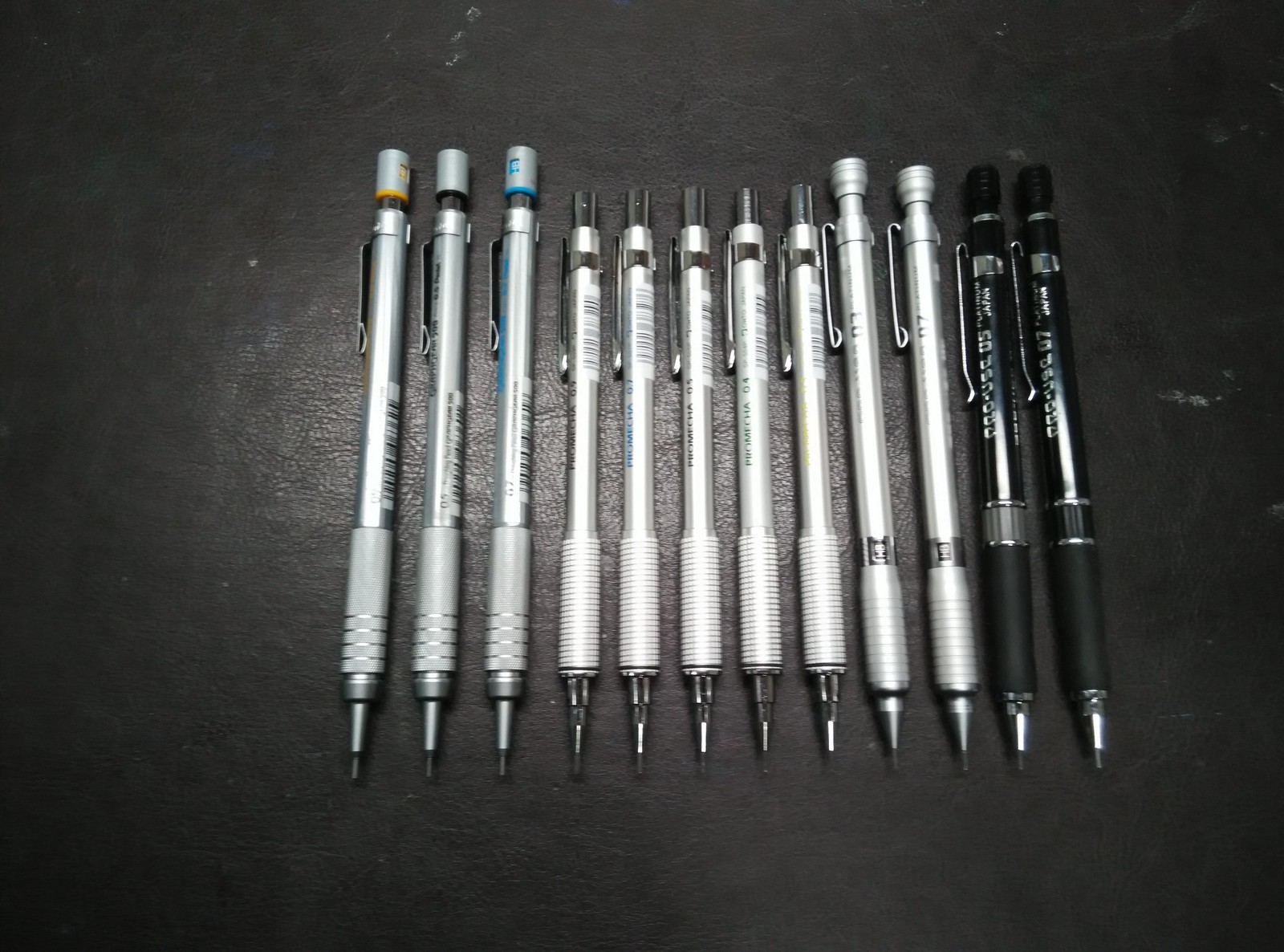In this image, twelve mechanical pencils and pens are meticulously arranged in a single row against a black, textured backdrop with a shiny, leathery appearance. The lineup presents a mix of heights, though all the tips are meticulously aligned. Starting from the left, the first three pens are tall and silver-toned with colored caps in yellow, white, and blue. Following these are five identical silver-toned pens with white striped grips, showcasing uniformity in their streamlined design. Next, two more pens with a silver-tone grip and slightly flared tops sit side by side, maintaining the metallic theme. Finally, the last two pens are distinguished by their matte black color, featuring silver writing and links that stand out against the dark finish. Each pen includes a silver-tone pocket clip, adding both functionality and a touch of elegance. The overhead lighting casts a gentle reflection on the sleek surfaces, enhancing the visual appeal.